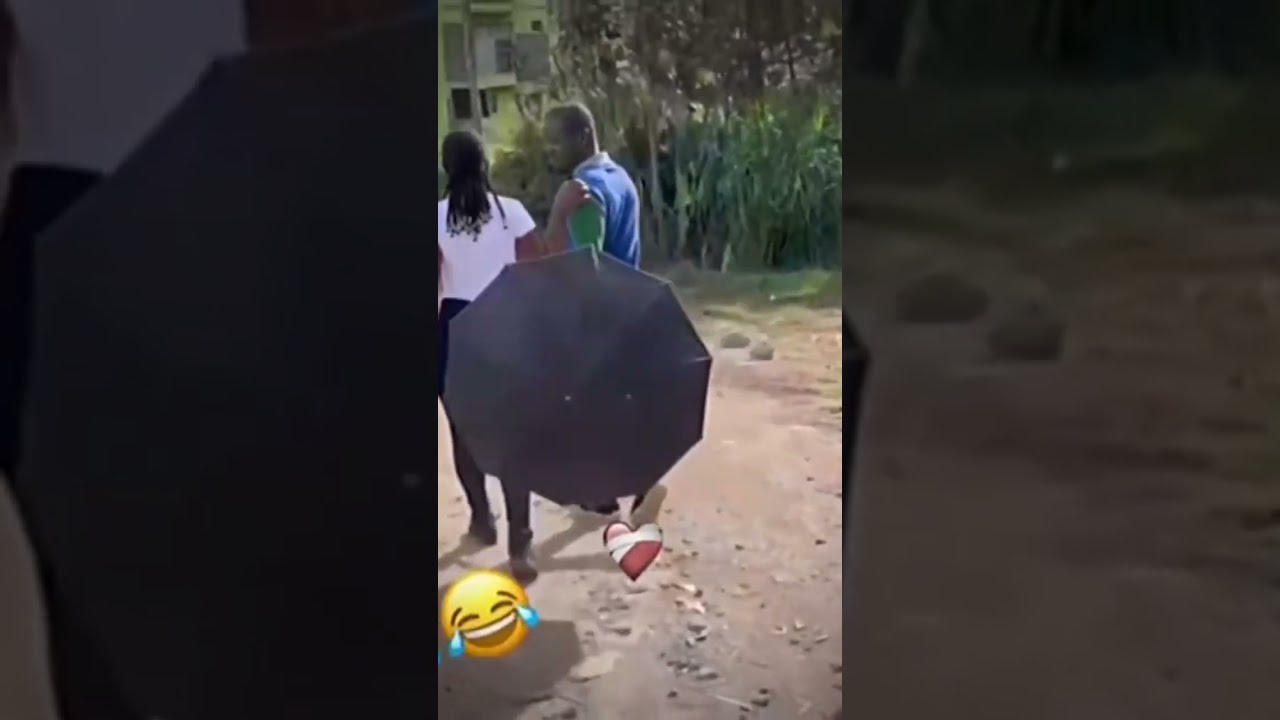In the center of the image, there's a scene featuring a black man and woman walking together on a dirt road or pathway, both partially obscured by a large, open black umbrella they are carrying, which covers the lower halves of their bodies. The man is on the right, wearing a blue shirt with green sleeves and a white collar, while the woman on the left has long braided black hair, a white shirt, and blue shorts. A yellow laughing emoji with blue tears hovers below her. They are positioned slightly to the left of the vertical, rectangular frame which is in sharp focus. Surrounding this central scene is a dimly lit, zoomed-in version of the same image, offset and tinged with dark colors. In the background, there are trees and shrubbery with a yellow building partially visible to the left.